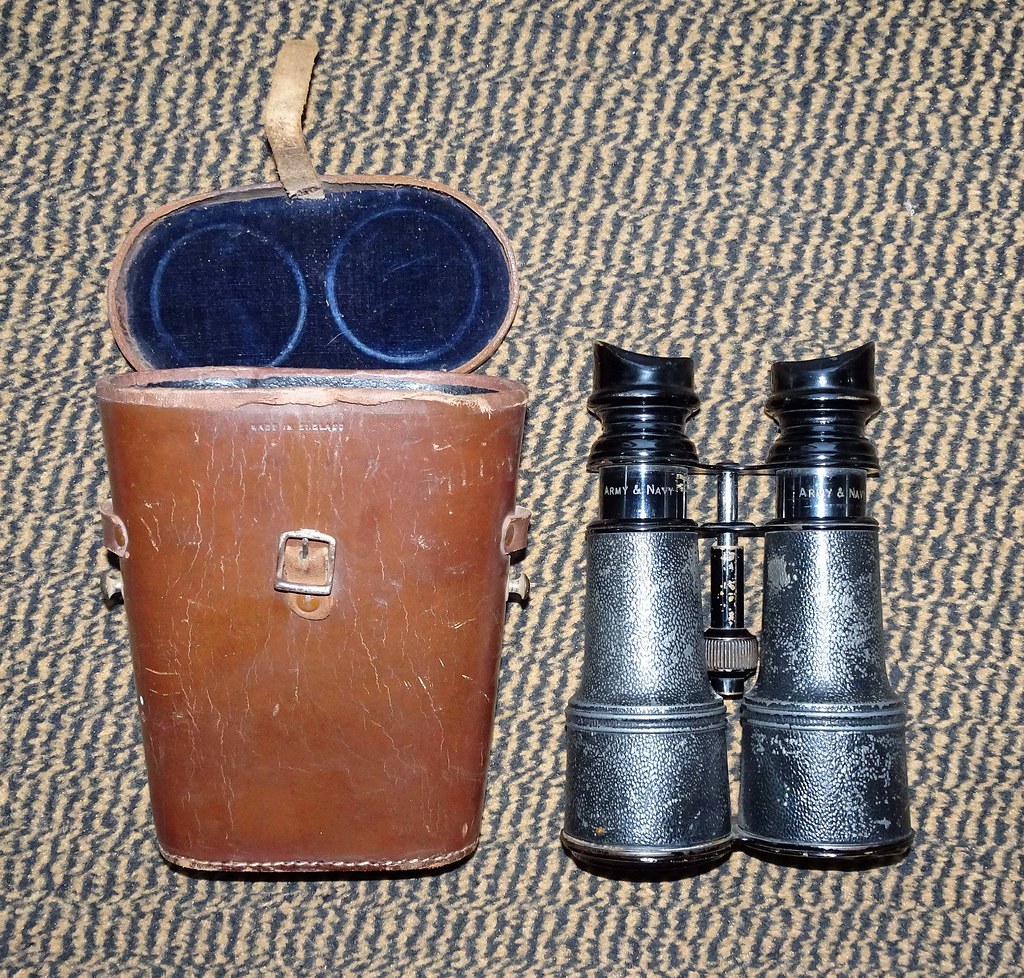This color photograph captures a small, antique pair of binoculars alongside their carrying case displayed on a blue and beige striped carpet. On the left, the brown leather carrying case is shown, its cover open to reveal a black velvet interior. The exterior is cracked with age, with a silver buckle on the front and loops for straps on the sides. The top of the case features small embossed gold text that reads "Made in England." To the right are the binoculars, predominantly black with textured grips near the lenses and shiny eyepieces. They have aged, revealing a grayish metallic color underneath. White text on either side near the eye ports states "Army and Navy."